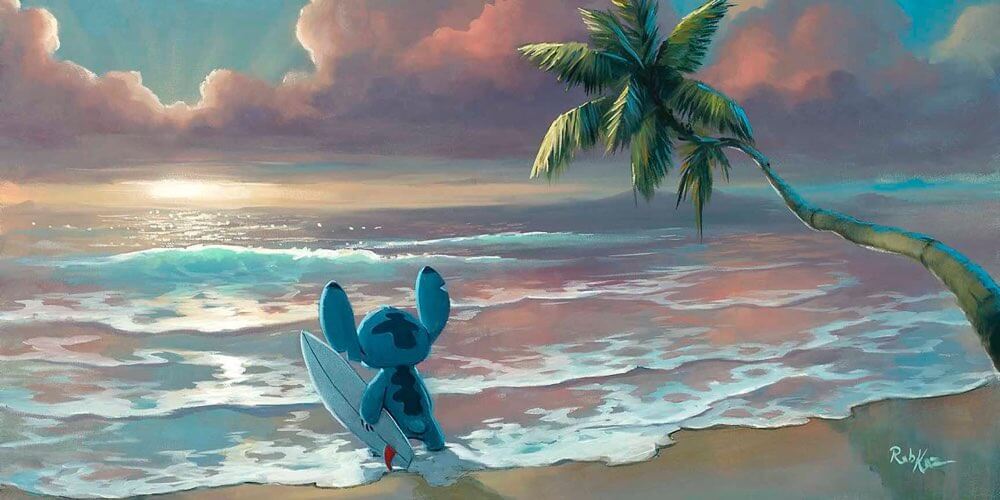The image is a detailed illustration of a serene beach scene, featuring vibrant pastel colors such as light blue, purple, gray, pink, and white blending harmoniously together. The sky is a rich blue adorned with reddish clouds that cast a warm hue over the calm ocean waters below. In the center of the horizon, the sun hovers, adding to the tranquil atmosphere. Small, gentle waves with white foam lap against the sandy shore. To the right, a crooked green palm tree leans over the beach.

At the bottom center of the illustration, the blue cartoon character Stitch from the animated series "Lilo and Stitch" is depicted from behind, walking towards the ocean while holding a small white surfboard under his left arm. His large ears stick out prominently, reflecting his unique and recognizable design. The artist's signature appears in white in the bottom right corner of the image, adding a personal touch to this charming and peaceful beach scene.